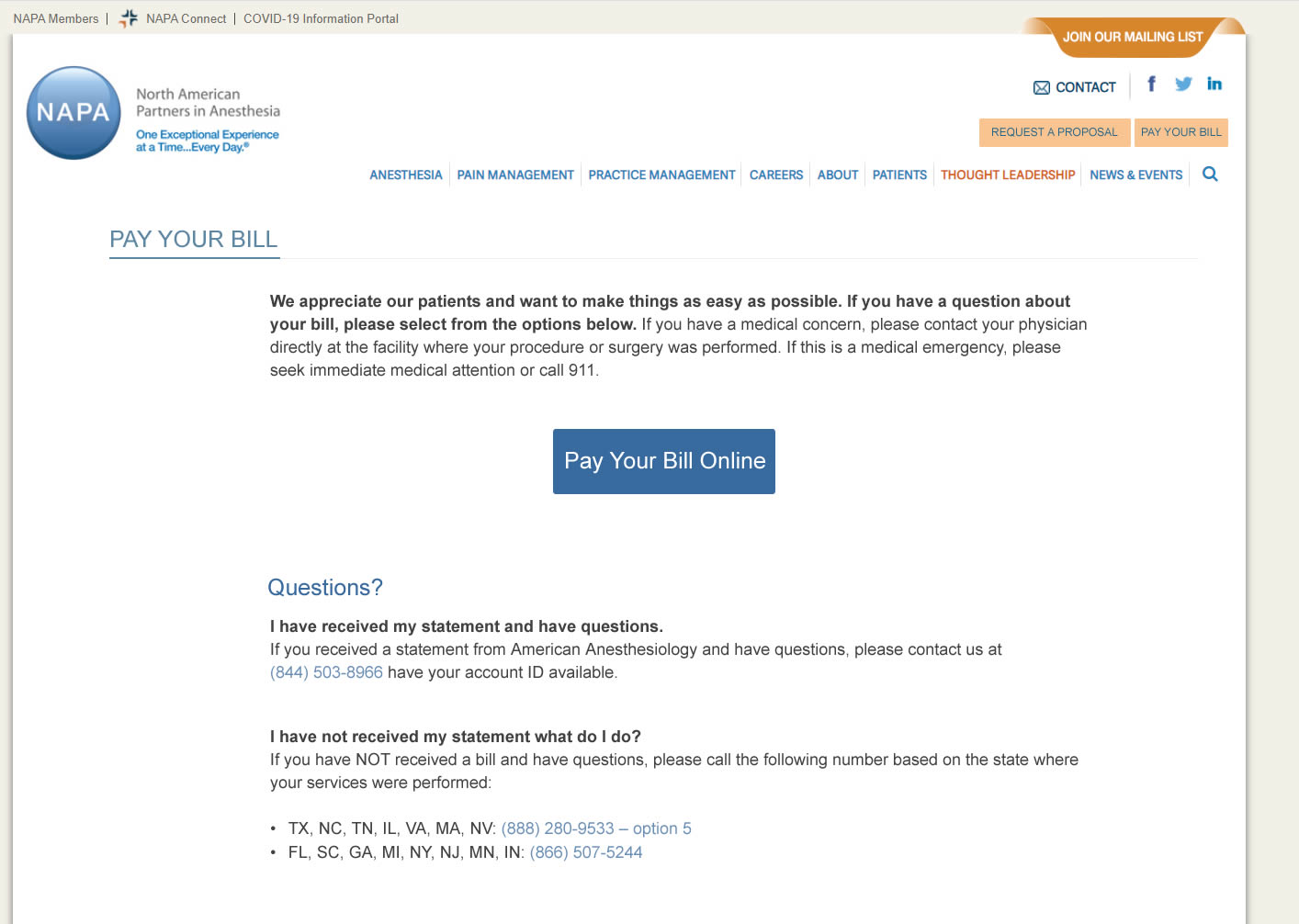This detailed and descriptive caption paints a clear picture of the webpage's layout and content:

---

This image showcases a screenshot of a web page featuring a beige border at the top and right side. Positioned in the upper left corner on this beige border, the text "NAPA Members, NAPA Connect, COVID-19 Information Portal" is written in black font. Below this, on a crisp white background, a blue circle is situated in the upper left corner with the acronym "NAPA" in white font. Adjacent to this, the black text reads "North American Partners in Anesthesia," and beneath it, the slogan "One Exceptional Experience at a Time... Everyday™," is presented in blue font.

In the upper right corner of the page, a small orange banner with white font invites visitors to "Join Our Mailing List." Beneath this banner, an envelope icon labeled "Contact" is accompanied by icons for Facebook, Twitter, and Instagram, providing quick access to their social media platforms.

Further down, two light orange buttons with blue font offer options to "Request a Proposal" and "Pay Your Bill." Below these buttons, the webpage features a sitemap with links categorized under "Anesthesia, Pain Management, Practice Management, Careers, About, Patients, Thought Leadership, News, and Events."

---

This caption details the visual elements and text on the webpage in a structured manner.